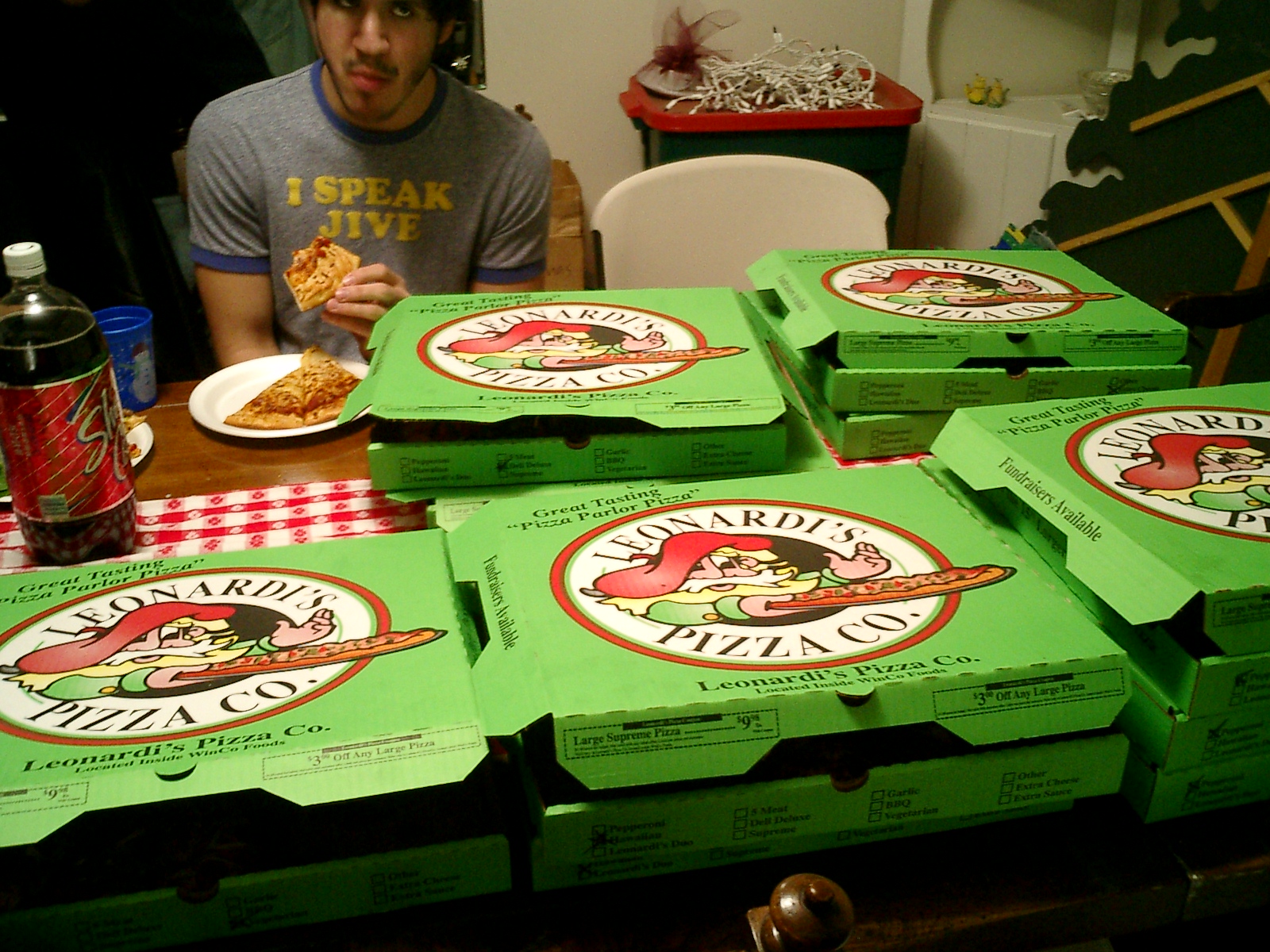In this horizontal photo, we are taken inside what appears to be a kitchen with tan walls and green containers in the background, adorned with some Christmas lights. The focal point is a young man of possibly Native American or Latino descent, sitting at a wooden table covered with a red and white checkered tablecloth. He's wearing a gray shirt with blue trim around the collar and sleeves, which bears the phrase "I speak jive" in yellow capital letters. The man has a mustache and sideburns, and is holding a half-eaten slice of pizza in his left hand. In front of him, there is a white paper plate with more pizza slices, and a blue cup featuring a snowman design. Beside the cup is a large bottle of cola with a red label and white cap. Scattered around the table are over a dozen light green pizza boxes, stacked in two layers. These boxes are from Leonardo's Pizza Company, each featuring a cartoon logo of a man named Leonardo, who is depicted with a red beanie, a beard, and a green outfit, holding a pizza in his right hand. In the background, there is a wastebasket with Christmas lights on top, and an empty white chair next to the table.